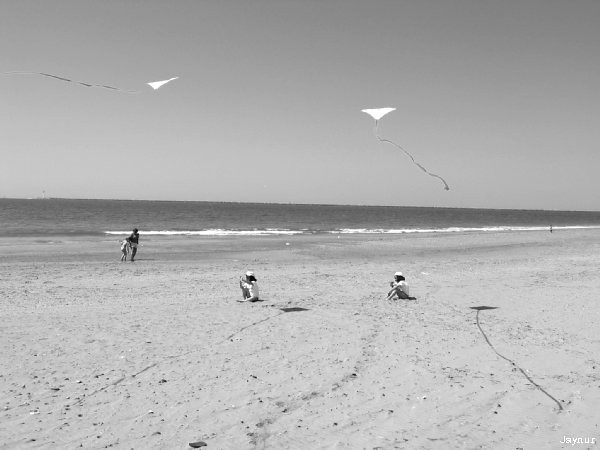A black-and-white photograph captures a serene beach scene with a wide expanse of sandy shore and a calm ocean in the background. The sky is cloudless and evenly toned. Two plain, white kites, potentially with streamers, float in the sky, casting distinct shadows on the textured sand below. In the left part of the image, a distant adult walks alongside a small child near the tranquil shoreline. Towards the center of the frame, two children, dressed similarly in white hats, white shirts, and shorts, sit on the sand, appearing to hold the kites above them, though their strings are not visible. The ocean forms a narrow, calm strip along the horizon, where a small indistinct figure, possibly a ship or lighthouse, can be seen to the far left. The bottom right corner of the photo bears a white watermark reading “Janus” or possibly "Jane Ewer," indicating the photographer’s signature.